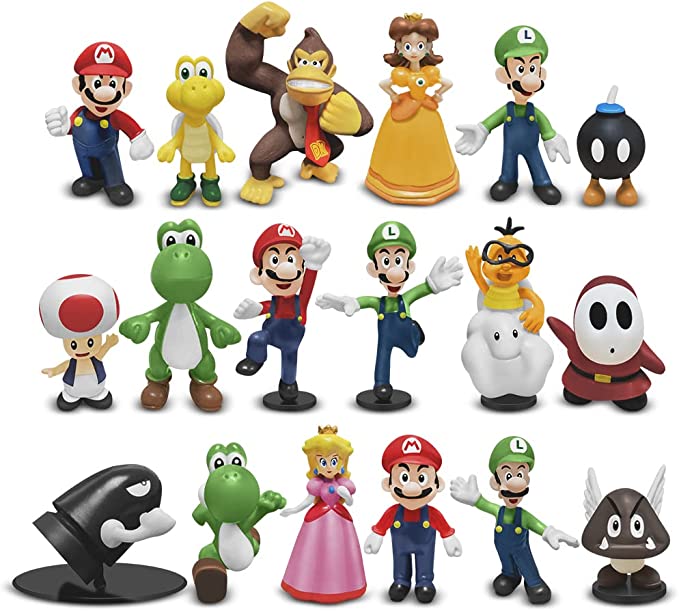The image features a collection of Super Mario Brothers character figurines organized into three rows against a plain white background. Each row displays different characters in unique poses, showcasing a variety of beloved figures from the franchise.

In the top row, from left to right, we see:
1. Mario striking a strong pose with his fist by his side.
2. A yellow Yoshi figurine standing upright.
3. Donkey Kong making a triumphant fist pump.
4. Princess Daisy looking forward with her arms forming fists by her waist.
5. Luigi with an expression of shock and his arms positioned in a questioning manner.
6. A Bob-omb with feet, poised at the ready.

The middle row features:
1. Toad, the mushroom character, smiling cheerfully.
2. Green Yoshi standing upright.
3. Super Mario standing on one leg, punching upward.
4. Luigi with his arms out to the side, balancing on one leg.
5. Lakitu, a turtle riding on a cloud.
6. Shy Guy, a small figure in a red robe with a white mask, black eyes, and a small black mouth.

In the bottom row, from left to right, are:
1. Bullet Bill, a black bullet with an eye and a white arm.
2. Green Yoshi depicted in a running motion.
3. Princess Peach with blonde hair, wearing her signature pink dress and crown.
4. Mario, once again, standing with his arms out to the side.
5. Luigi, having one arm up in the air and the other down to the left.
6. A Para-Koopa, a black and white colored Koopa with wings.

This detailed arrangement provides a vibrant showcase of collectible figurines, each character captured in signature poses indicative of their personality and role in the Super Mario universe.